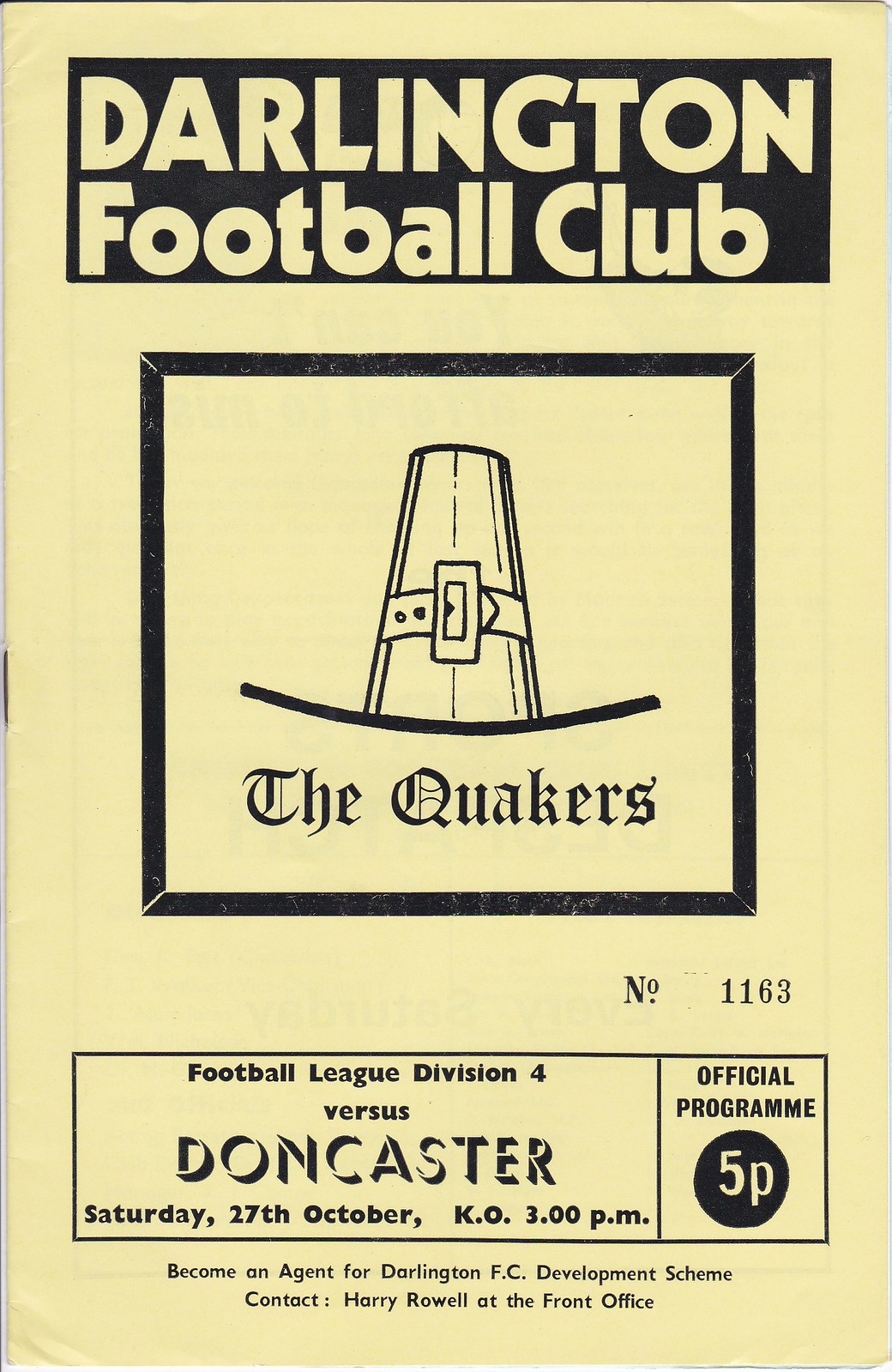The cover page of the football official program features a yellow background with black text, creating a striking yellow-black design. At the top, it reads "Darlington Football Club" in black font. Central to the design is a black-bordered box containing an image of a Quaker hat, symbolizing the team. Beneath the hat, the text "The Quakers" is prominently displayed. Further down, it reads "number 1163." Below this, in a horizontal box, the details of the match are presented: "Football League Division Four versus Doncaster. Saturday, 27th October, K.O. 3 p.m." Additionally, it invites readers to "Become an agent for the Darlington FC Development Scheme" and provides contact details: "Contact Harry Rowell at the front office." The bottom of the cover states that this is the "Official Program, priced at 5p."